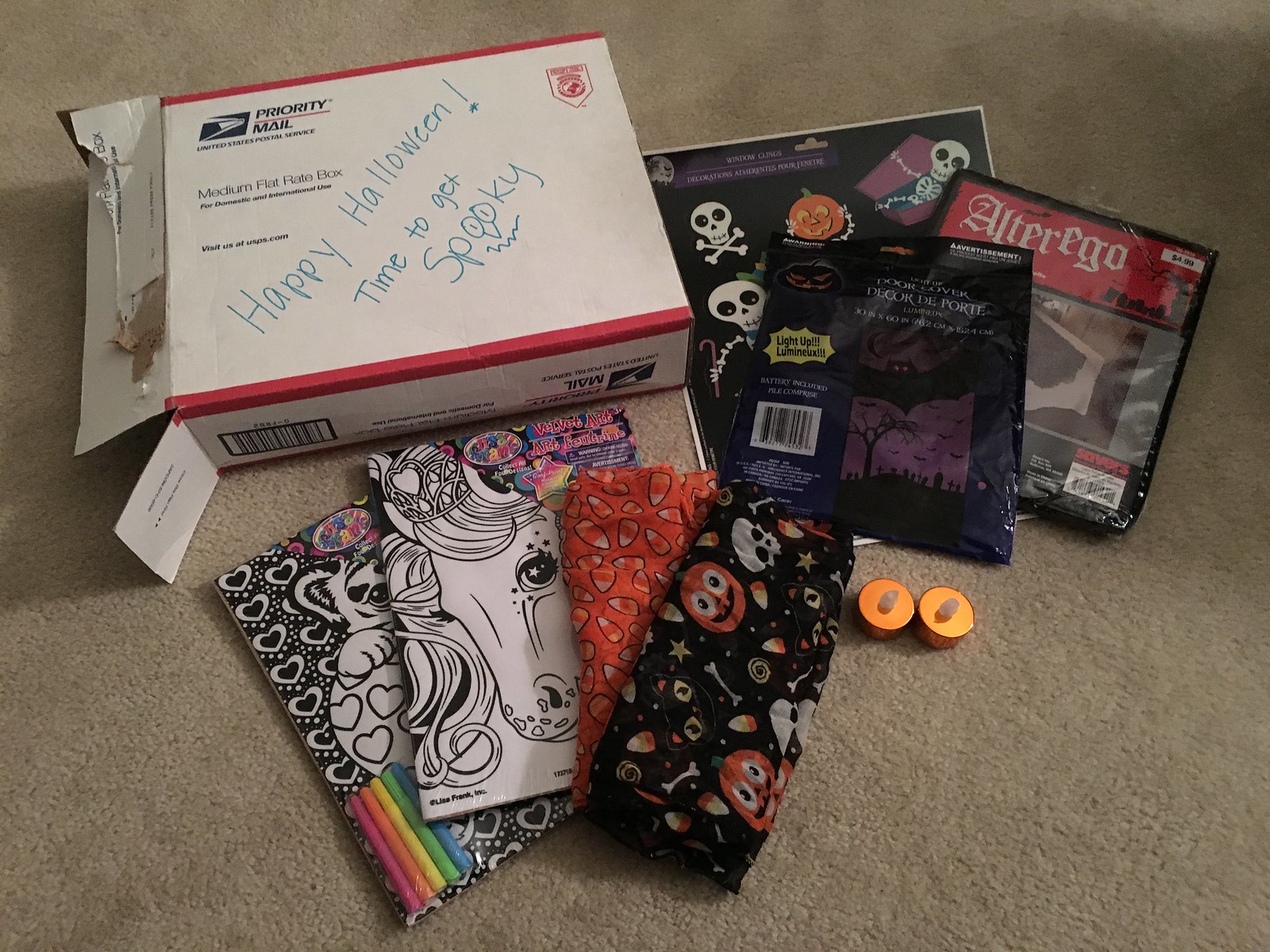The image is a detailed photo of a Halloween-themed care package on a white rug. On the left upper portion of the image, there's a U.S. Postal Service Priority Mail box that has been ripped open. The box is medium flat-rate and has handwritten text diagonally across it, reading "Happy Halloween, time to get spooky!" with the double O's in 'spooky' creatively illustrated to resemble eyes with a beak below them. 

Inside and around the open box are various Halloween-themed items. Notably, there are multiple packages featuring Halloween motifs such as skeletons and pumpkins. There's a bandana adorned with pumpkins and another package with decals of skeleton heads. Additionally, there is a coloring book with heart designs and a Pegasus on the cover, and another coloring package containing a horse’s head illustration in black on a white background. Also visible are two small tan items, possibly earplugs, on the surface near the packages. 

In the upper right of the scene is a package labeled "Alter Ego," likely part of a Halloween costume set. There are also items that look like Halloween loot bags in orange and black, and a booklet with a black pamphlet featuring skeleton designs. The overall assortment exudes a festive, spooky atmosphere, ready for Halloween celebrations.